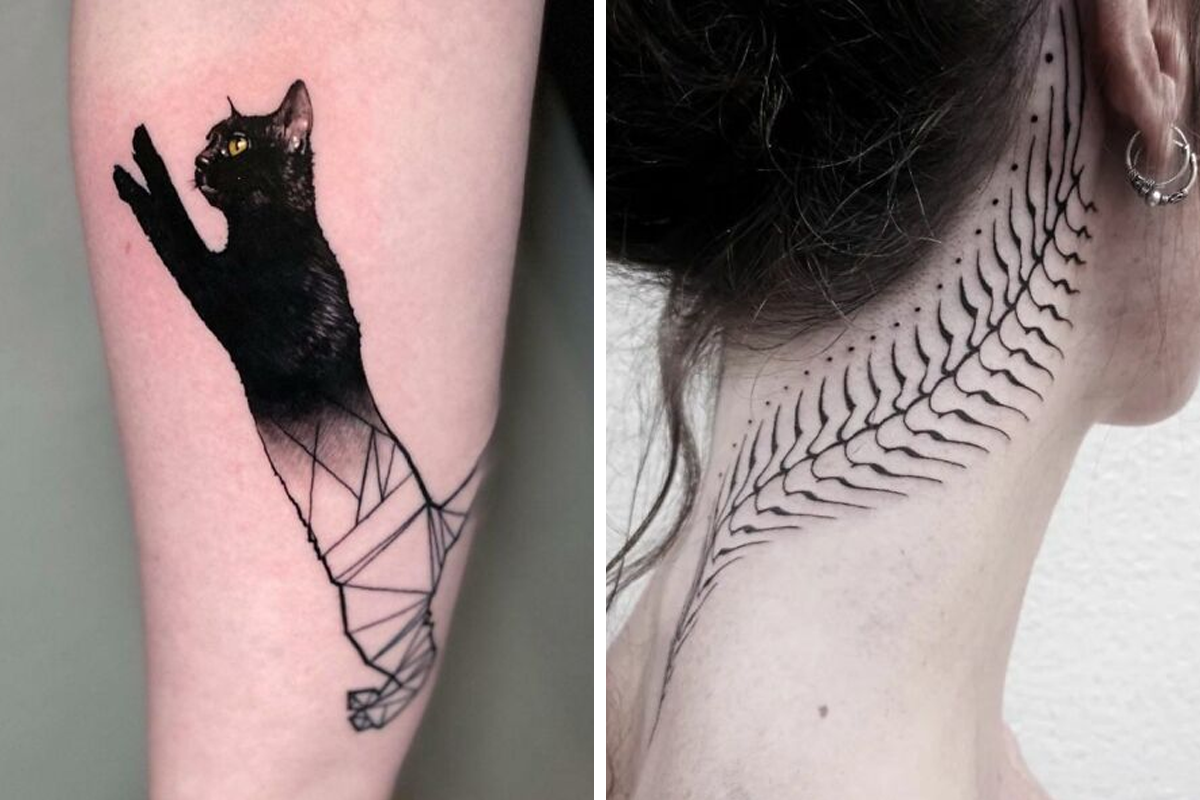The image showcases two distinct tattoos on a person's body. On the left side of the photograph, a detailed tattoo of a black cat with striking green eyes is featured on someone's inner forearm. The cat is depicted with its paws raised above its head, as if leaping. The top half of the cat is solidly black, transitioning into a crisscross stencil design toward the lower half. The cat faces left, with its black tail curling elegantly behind it. 

On the right side of the image, the back of a woman's neck is visible, accentuated by her updo, which reveals a detailed leaf or fern-like tattoo. This tattoo starts at the back of her ear and extends gracefully down her neck, tapering off slightly onto her upper back. The design features a central stem with delicate, swirling branches reminiscent of a feather or fern fronds. Several small dots embellish the ends of these branches, enhancing the intricate pattern. The woman is also wearing two hoop earrings in her right ear, further drawing attention to the tattoo. The photograph is horizontal, allowing a thorough view of both striking tattoos.